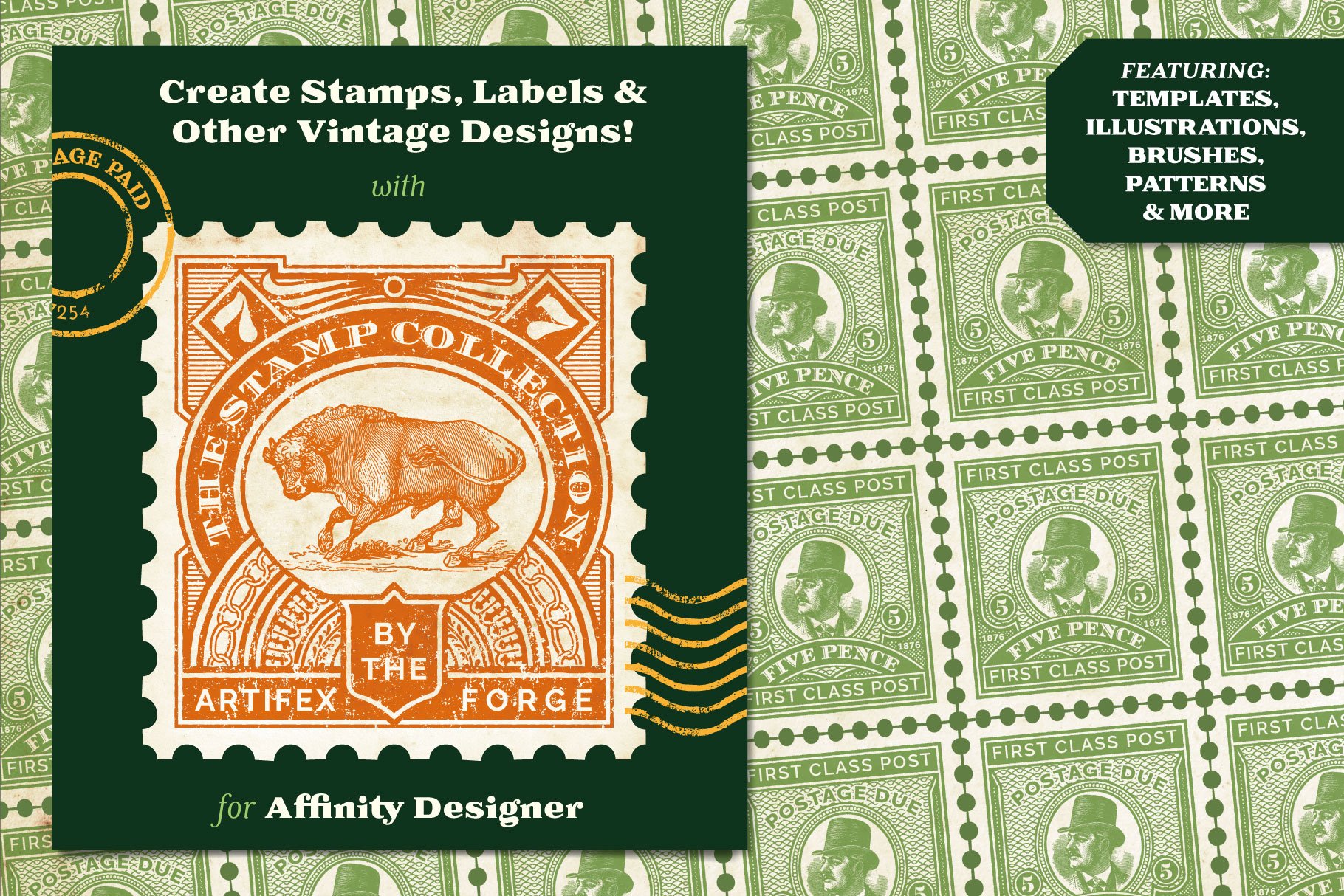This advertisement showcases the creative possibilities offered by Affinity Designer with a focus on vintage-style stamp designs. The background is adorned with multiple green, old-fashioned stamps, each bearing the repetitive text "first class post" and "post is due, five pence." Central to the image is a detailed orange stamp, prominently placed within a large green square on the left side. This stamp, titled "Stamp Collection Artifacts by the Artifex Forge," features intricate designs, including a buffalo in the middle of a white-outlined circle, flanked by the number sevens and a gold cancellation mark. Above this stamp, a tagline reads: "Create stamps, labels, and other vintage designs with Affinity Designer." Another focal point is a gentleman in a distinguished top hat and Edwardian attire seamlessly integrated into the background stamps. The upper right corner of the image emphasizes the application's versatility with the text: "Featuring templates, illustrations, brushes, patterns, and more."